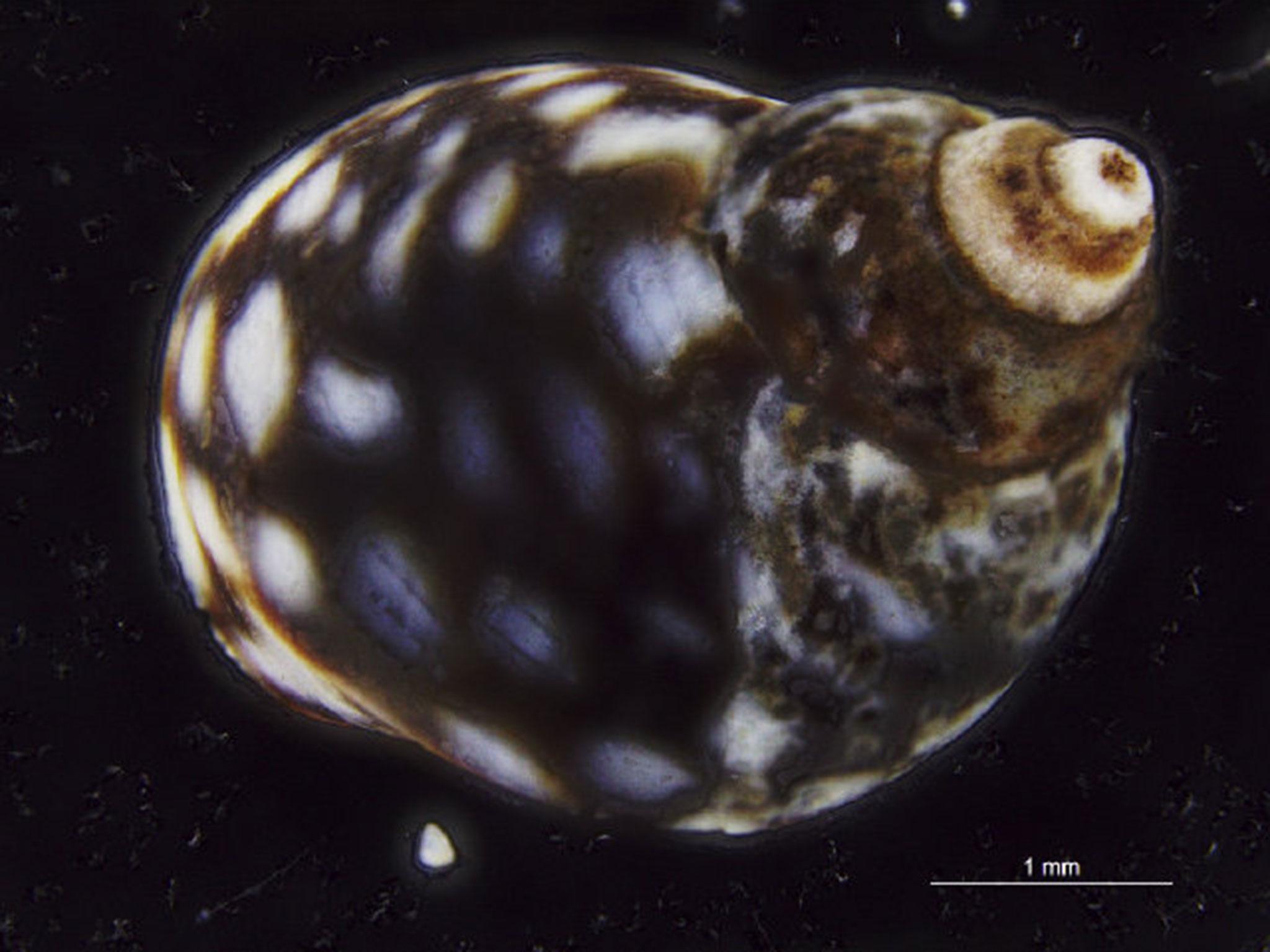The image features a detailed, magnified view of a small, rounded shell, resembling a snail or hermit crab shell. The shell is dark brown with white splotches interspersed with black stripes. It has a smooth, unbroken surface that spirals into a pronounced curl at the end, transitioning from brown to a cream color where the curl tightens. Positioned against a black background, the image reveals scattered brown dust-like particles, contributing to the underwater ambiance suggested by the dark backdrop. In the upper right corner of the shell, the white areas are bordered by brown. The bottom section of the shell showcases a pattern of white and black specks of varying sizes. The image includes a white scale bar labeled "1mm" in the bottom right corner, signifying the magnified nature of the photograph and suggesting the shell's true small size.